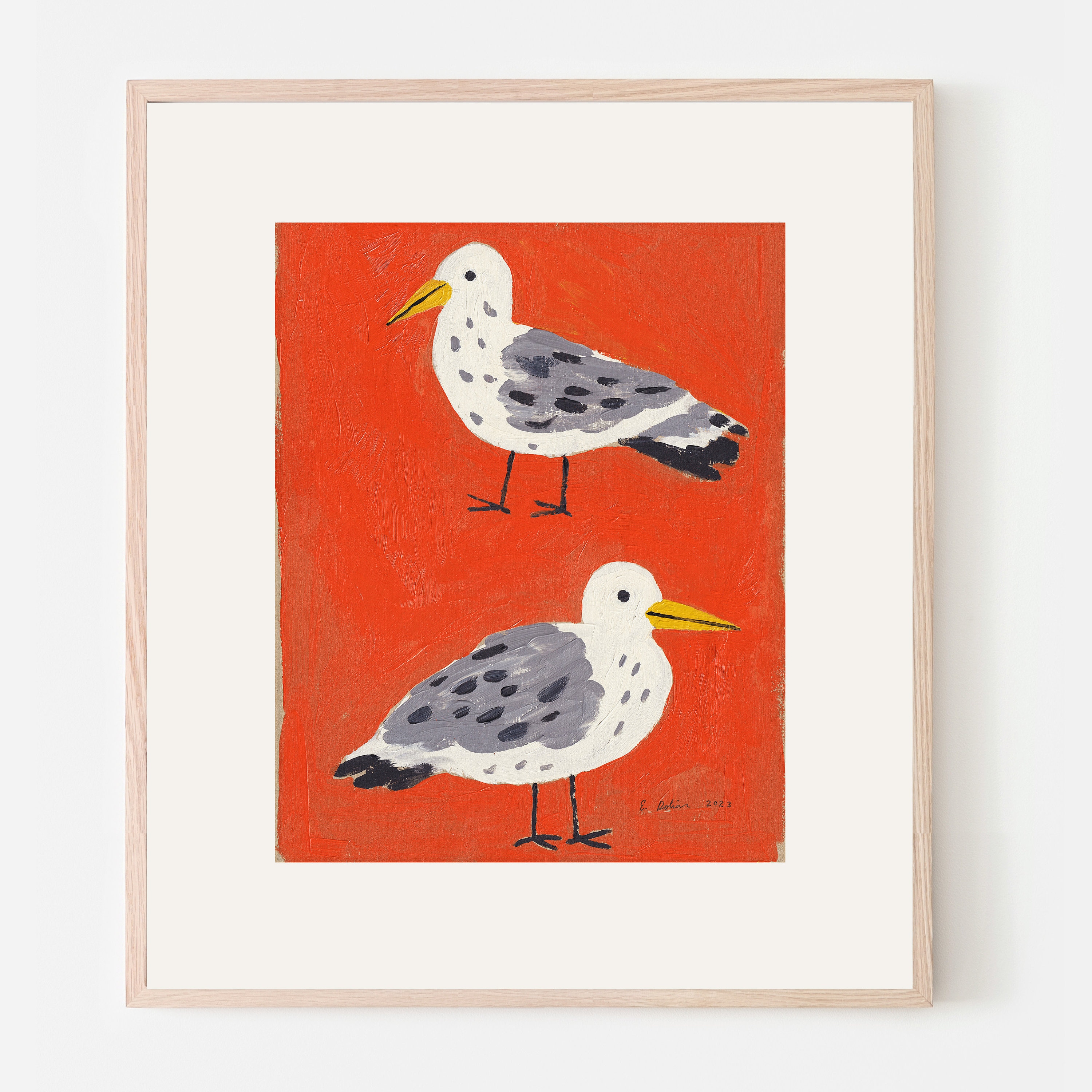This image depicts a minimalist painting of two seagulls, framed and hanging on a white wall. The birds are rendered in a two-dimensional style on a red-orange background, with visible painted texture. The artwork is housed in a thin light walnut or beige wooden frame with a thick white matte border. The seagull at the top faces left, while the one at the bottom looks right; both birds feature white heads and bellies, gray wing feathers with black accents, and tails that blend gray, white, and black. They also have characteristic yellow beaks and thin black legs. The bottom right corner of the painting shows the artist's initials and date in small black text.